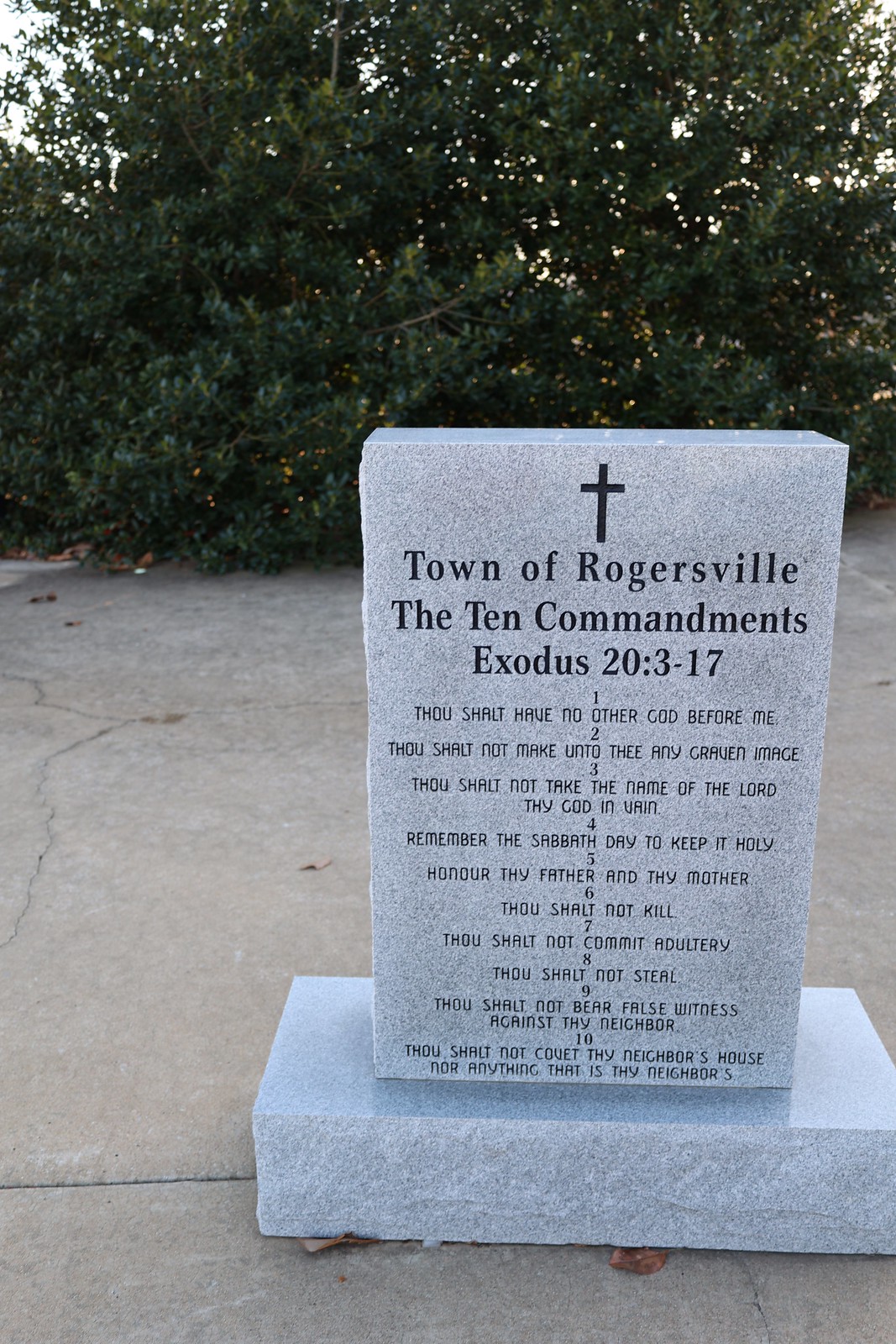This photograph captures a detailed marble marker set against a backdrop of lush greenery. The marker is light gray, almost bluish in hue, and positioned on a rough-edged marble pedestal, which rests upon a concrete surface reminiscent of an aged sidewalk or driveway, featuring noticeable cracks. At the top center of the marker, there is a prominent black cross. Below the cross, inscribed in capital letters, are the words "Town of Rogersville" and a reference to "Exodus 20:3-17." The main body of the marker meticulously lists the Ten Commandments, each commandment numbered from one through ten, with the text carved in a distinctive, yet somewhat indiscernible font. While it visually resembles a gravestone, it is, in fact, a dignified memorial plaque dedicated to the Ten Commandments, embodying both historical and religious significance.